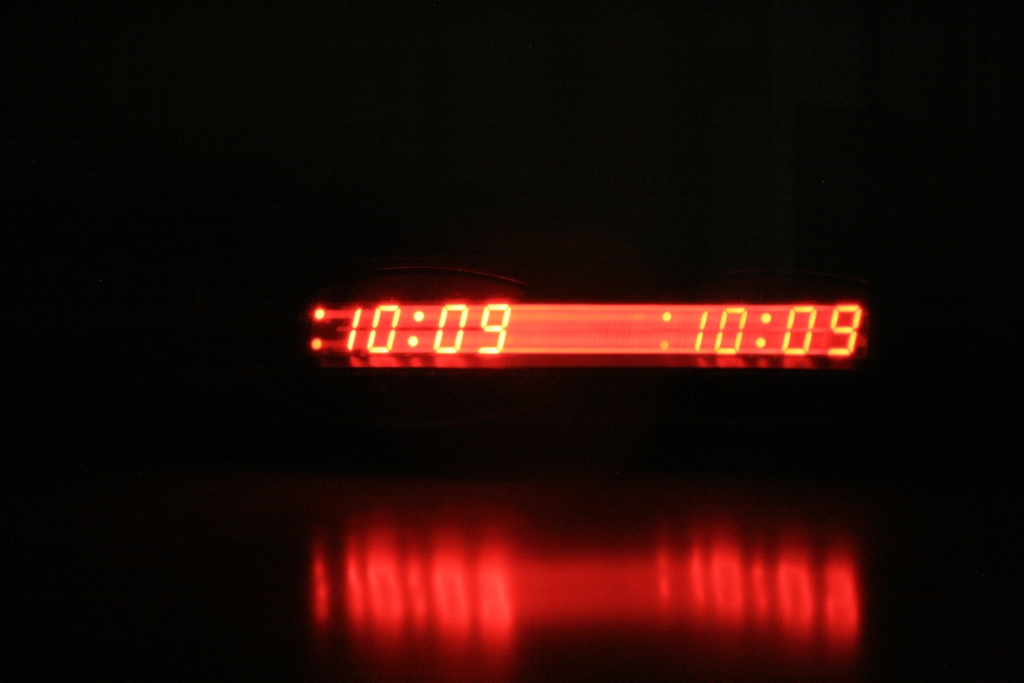The image predominantly features a deep black background, accentuating the illuminated elements within. At the center is the vibrant face of a clock, characterized by a rich red coloration. The numerals and symbols on the clock are rendered in a striking bright yellow, clearly displaying the time as 10:09. To the right of the clock face, there is a noticeable reflection, which also reads 10:09. However, this reflection appears darker and slightly blurred, creating a subtle contrast in clarity and color. Below this, another reflection of the numbers "10:09" can be seen, but this time in an even darker, more muted red hue and significantly more blurred, making it less legible. Despite these illuminating details, the surrounding area of the image remains enveloped in a pitch-black void, emphasizing the stark brightness and reflective qualities of the clock's face and its mirrored counterparts.